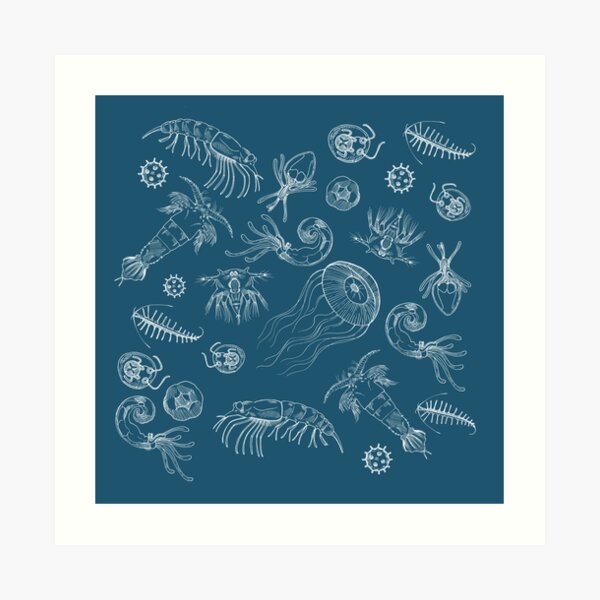The image features a detailed white sketch of various sea creatures on a blue background, resembling marine life you might find in the ocean. At the center of the picture, a menagerie of approximately 25 different creatures is intricately drawn, with a pale, almost translucent appearance that allows you to see through them like skeletons. Among the identifiable creatures are jellyfish, shrimp, krill, and something resembling a small crawfish, characterized by long feelers and appendages. Additionally, there are numerous enigmatic figures, including circular forms with dots and fibers emanating from their perimeters, suggesting some kind of underwater organisms or microscopic beings. The entire blue square is densely populated with these assorted marine drawings, each showcasing a unique aspect of oceanic life.